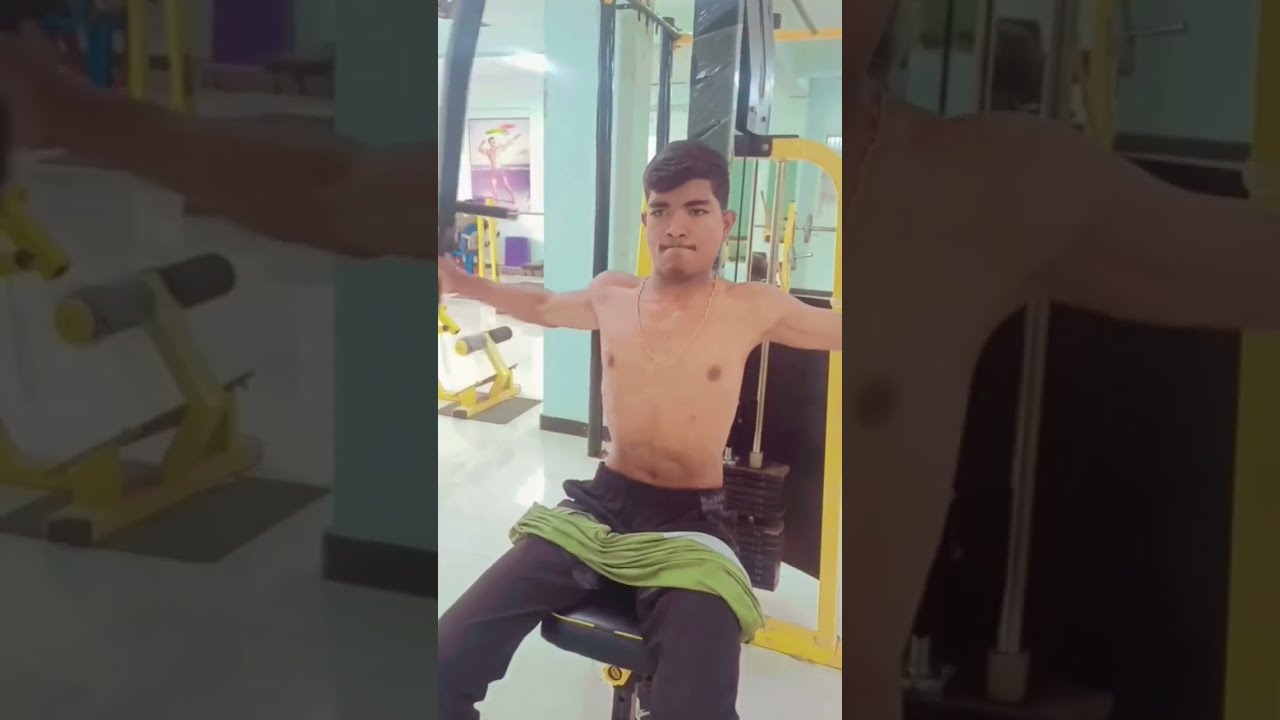In this detailed high-definition photo, a young Filipino man is working out intensely at the gym, which features light green walls and yellow equipment, reminiscent of a Planet Fitness setting. He is seated on a chest fly machine, arms fully extended outwards, preparing to bring the handles together in front of him for a chest exercise. He is shirtless, revealing his lean physique and the gold chain around his neck. His green shirt is casually draped over his lap, and he is wearing long black sweatpants. His dark hair and features, including brown eyes and slightly darker skin, are highlighted under the gym's lighting. He has a grimace on his face, likely from the exertion of the workout, and appears to be holding his breath. The gym is empty behind him, emphasizing his solitary focus on the exercise. The overall image is tall and narrow like a cellphone photo, with faded close-ups on either side, showing detailed views of his extended arms and shoulders.